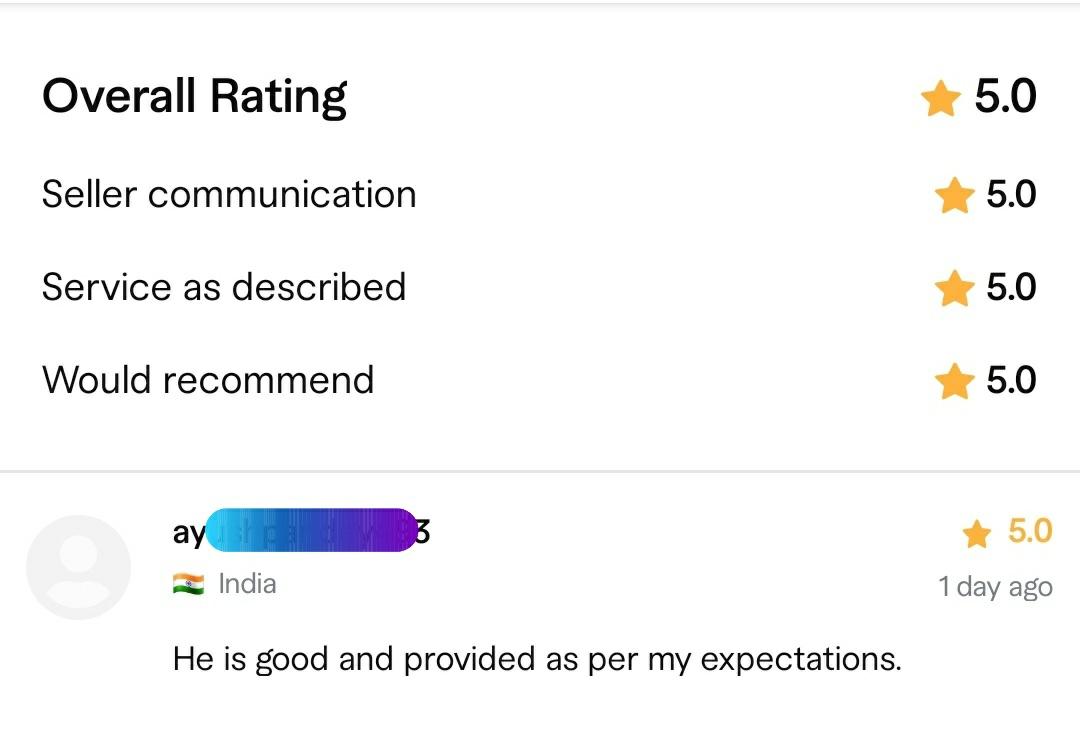This image is a screenshot of a user review on a service or website. The top section prominently displays an "Overall Rating," which is highlighted in bold black text. Adjacent to it on the right is a yellow star with a "5.0" rating, indicating a perfect score.

Below the overall rating, there are three subcategories, each followed by a yellow star and a "5.0" rating in black text, but in a slightly smaller and less bold font. These subcategories are:
1. "Seller Communication"
2. "Service as Described"
3. "Would Recommend"

The next section features a profile picture silhouette of a person. The accompanying name is obscured by a blue and purple bar. Below this, the user's country, "India," is specified next to a tricolor flag icon in red, white, and green. 

The review text reads, "He is good and provided as per my expectations," and is followed by an orange star with a "5.0" rating. At the bottom of the screenshot, the text "one day ago" appears in gray, indicating the recency of the review.